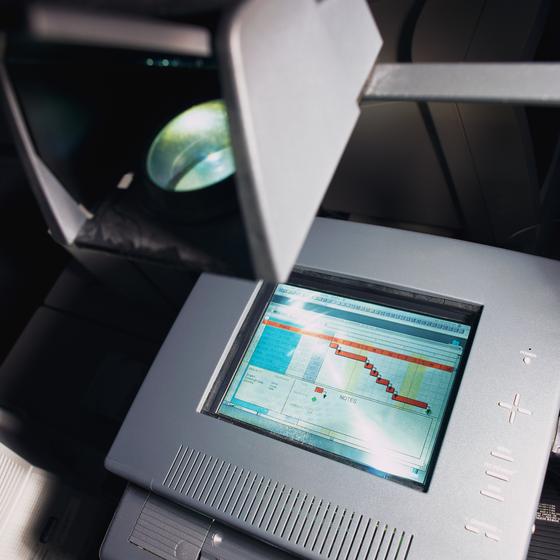In the center of this room, the photograph captures a sophisticated projection device encased in a gray, metallic housing. This device features a prominent glass lens at the top left corner from which a bright white or yellow light emanates, projecting onto a screen below. The screen, set on the bottom portion of the projector, displays a data visualization that includes colors like blue, red, yellow, and white, possibly showcasing a bar chart or other scientific graphic with a step-like pattern.

Adjacent to the screen, on the right side of the projector, are several control buttons arranged in a directional pad layout (left, right, up, down). Additionally, there are a couple of other buttons that seem to operate volume or similar functions. The details within the projection are intricate, suggesting the data is technical or scientific in nature.

The room setting and the device's streamlined design give the impression of advanced imagery technology, akin to a microscope or a high-tech media presentation system.